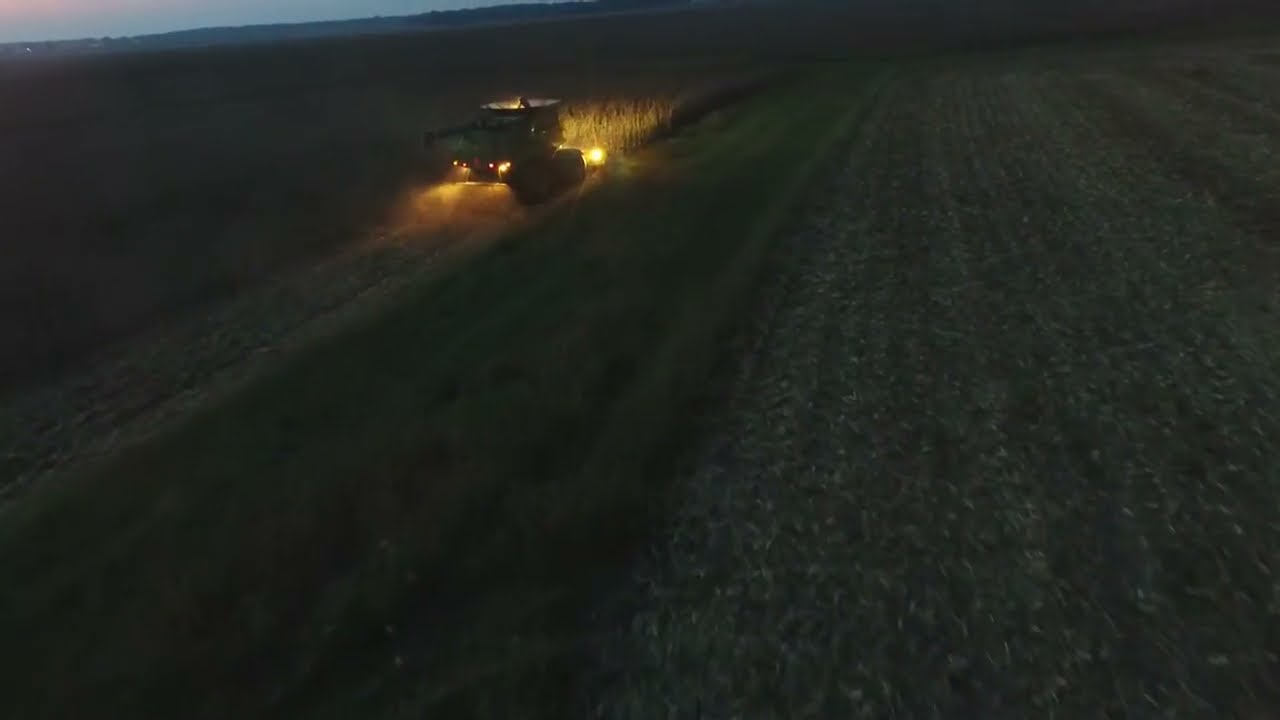In the image, a farmer is diligently working on his field, which is part of a farm, either very early in the morning or late at night, as indicated by the tractor's illuminated lights. The tractor, situated on the left-hand side and featuring large black tires and a green body with a rooftop that is either white or black, is actively harvesting crops. The field is divided, with part of it already harvested and the other part currently being worked on by the farmer. The harvested section appears brown and dirt-like, possibly indicating crops like corn or wheat. On the right side of the tractor, there's a strip of unharvested green crops. The background reveals some low-lying hills and a faint sky with a pinkish hue, suggesting a setting or rising sun. The scene is devoid of any text and encapsulates the hardworking nature of farm life.